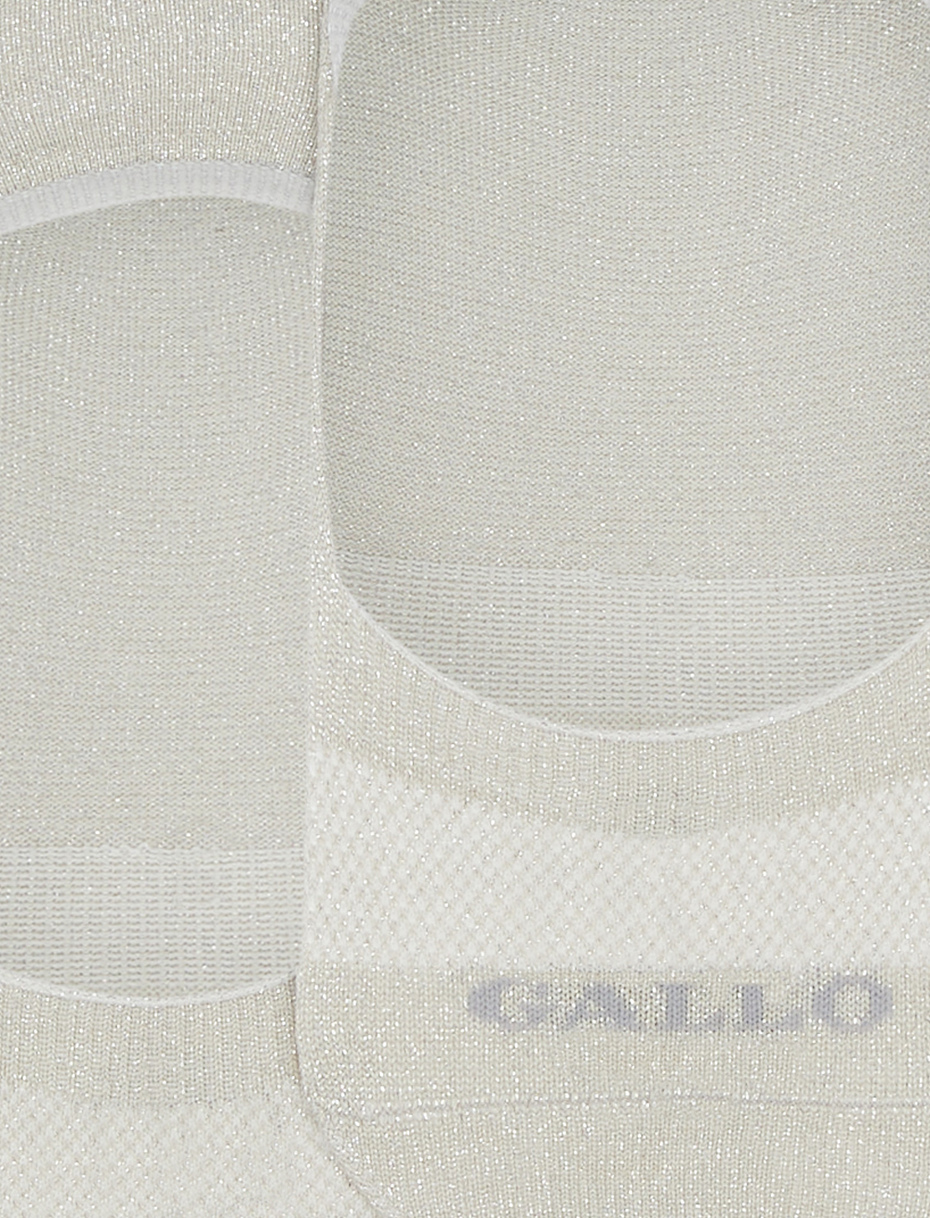A highly zoomed-in image captures two overlapped fabric objects, possibly socks or booties, laid flat. The objects exhibit a durable, textured, off-white cloth, suggesting a sturdy material similar to a tent fabric or knee brace. A vertical division, covering about 40% from left to right, hints at two distinct parts or pairs. Both items feature semi-circular patterns at the top, reminiscent of knee pads, and exhibit varying tan shades, from a darker sand color near the bottom to lighter hues closer to the opening. The fabric shows banding around key areas, like openings and edges, which adds to their garment-like appearance. The right object bears a slightly darker gray logo reading "Gallo" at the lower right, which is likely a brand name. The zoomed perspective limits the ability to see the full objects, leading to a guess that these are probably socks or slip-ons, potentially used in footwear, such as heels.